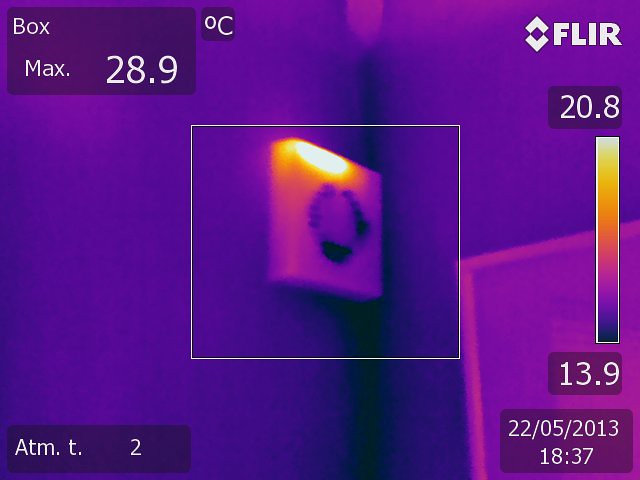The image features a square, white device mounted on a wall, captured in a purplish hue. The device resembles a temperature and pressure gauge, presenting various digital readings. Despite the image's blurriness, the gauge’s face seems to include a dial or circular display with numbers, further suggesting its measurement functions. In the upper left corner, the display reads "Box Max 28.9 degrees Centigrade," indicating the current temperature. The lower left corner shows "ATM2," likely representing atmospheric pressure. Additional numbers can be seen, hinting at other recorded parameters. The bottom right corner displays the date as "2205 2013."